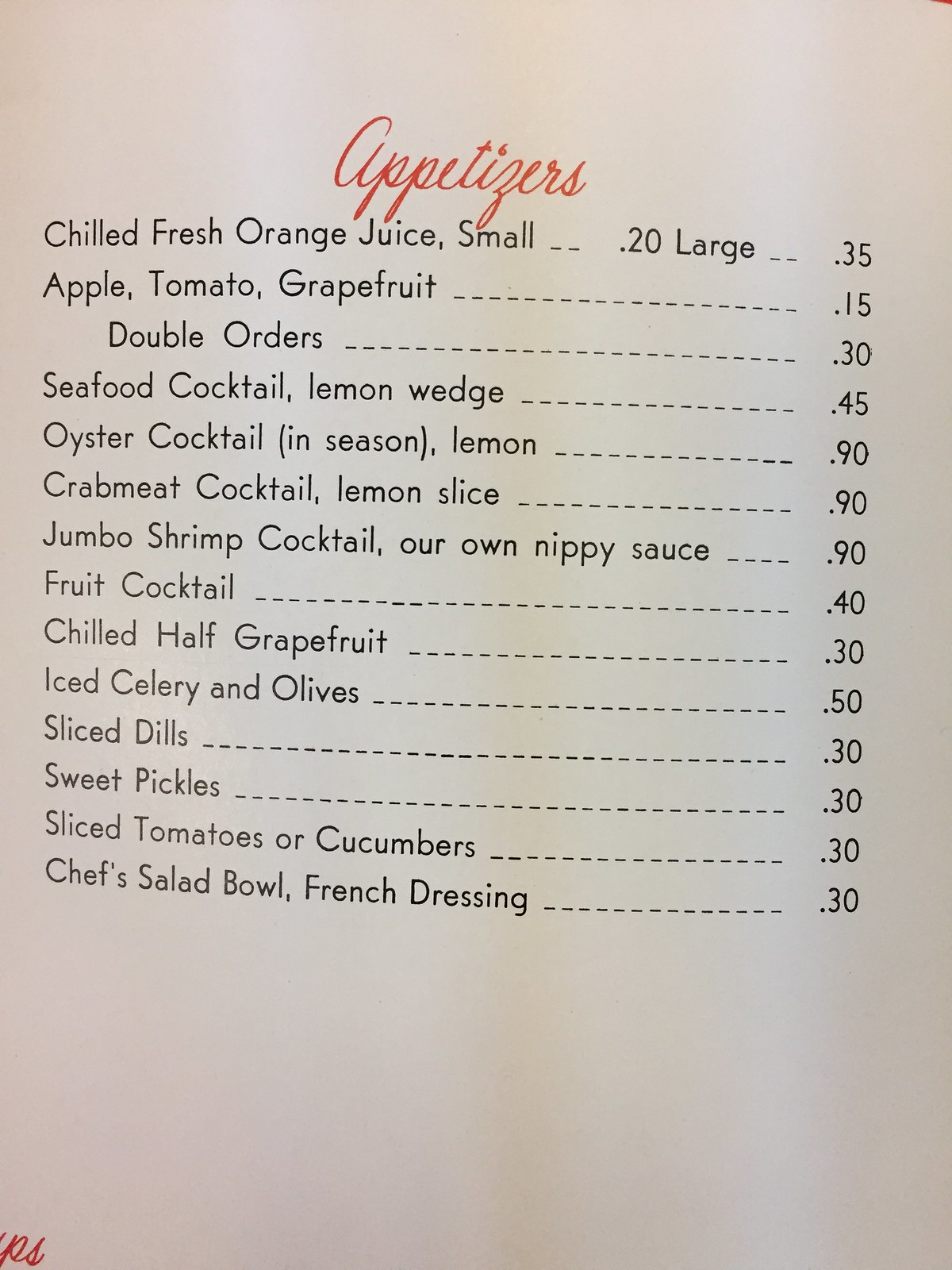Photograph capturing a section of a vintage menu page with distinct black and reddish lettering. In the bottom left corner, only the partial letters 'P' and 'S' are visible. The heading "Appetizers" is prominently displayed at the top in red. Beneath this heading, a clearly itemized list of appetizers is presented alongside their respective prices, albeit in an unspecified and seemingly minute denomination. 

The appetizers include:
- Chilled Fresh Orange Juice: Small $0.20, Large $0.35
- Apple, Tomato, or Grapefruit Juice: $0.15
- Double Orders: $0.30
- Seafood Cocktail with Lemon Wedge: $0.45
- Oyster Cocktail in Season with Lemon: $0.90
- Crabmeat Cocktail with Lemon Slice: $0.90
- Jumbo Shrimp Cocktail with House-Made Nippy Sauce: $0.90
- Fruit Cocktail: $0.40
- Chilled Half Grapefruit: $0.30
- Iced Celery and Olives: $0.50
- Sliced Dills: $0.30
- Sweet Pickles: $0.30
- Sliced Tomatoes or Cucumbers: $0.30
- Chef's Salad Bowl with French Dressing: $0.30